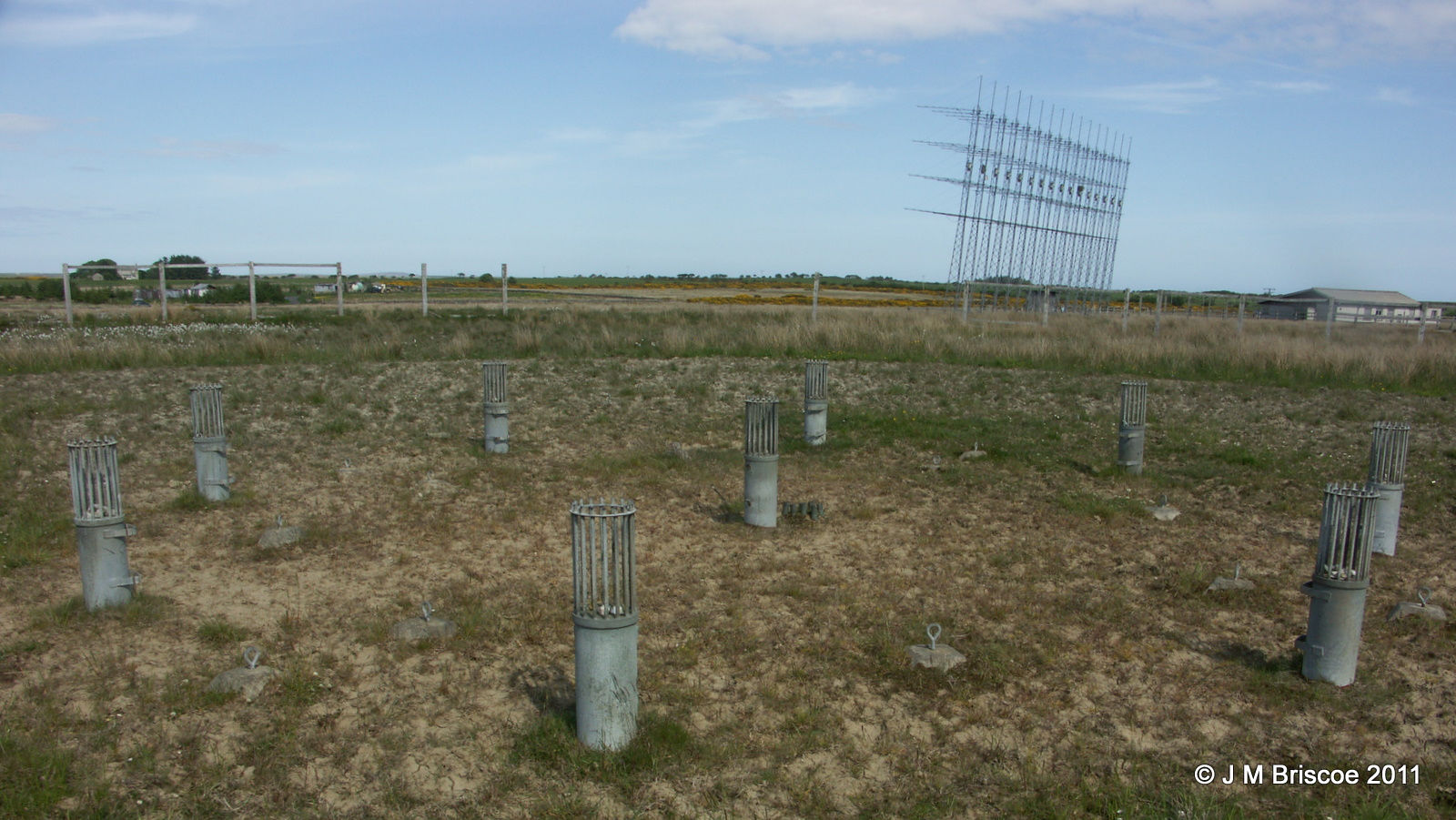The image depicts an open, sparsely grass-covered field with patches of dirt and green grass scattered throughout. Emerging from the ground are several conical metal structures with grated tops and solid bases, resembling pipes or possibly ventilation shafts. The field is bordered by a fence, beyond which lies another field and a square, gridded metal structure rising higher. In the background, a gigantic antenna towers over the scene, further emphasizing the utilitarian nature of the landscape. The sky is blue with some clouds, creating a calm atmosphere. On the right-hand side of the image, a few buildings can be seen, while two more are visible in the distance on the left. The horizon features a mix of foliage and possibly cars. Additionally, there are scattered concrete pillars in the foreground that appear half-built, adding to the industrial feel of the scene. Text at the bottom right reads, "Copyright JM Briscoe 2011 www.jamesbriscoe.com."